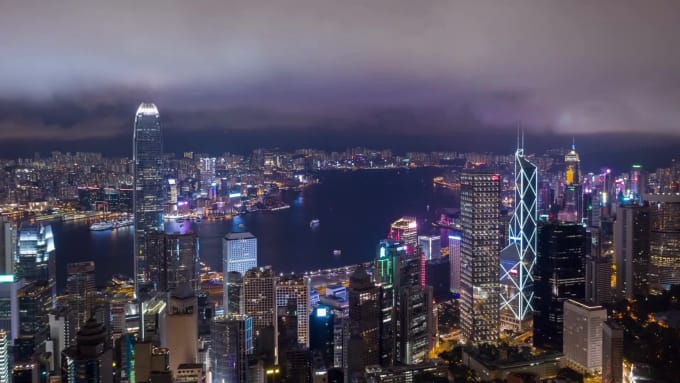This nighttime aerial image showcases the sprawling skyline of a major city, illuminated against a cloudy night sky. The scene features an array of towering skyscrapers adorned with a variety of colored lights—blue, green, pink, and glowing shades of gray—adding to the city's vibrant ambiance. The bustling cityscape is bisected by a winding river that runs from the left corner to the top middle of the image, dotted with boats gliding peacefully on its surface. Diffused clouds stretch across the sky, allowing glimpses of moonlight to cast a gentle glow over the entire landscape, contributing to a calm, serene atmosphere. The photo captures a highly urbanized area with a densely packed collection of buildings, creating a mesmerizing blend of architectural marvels and natural elements.